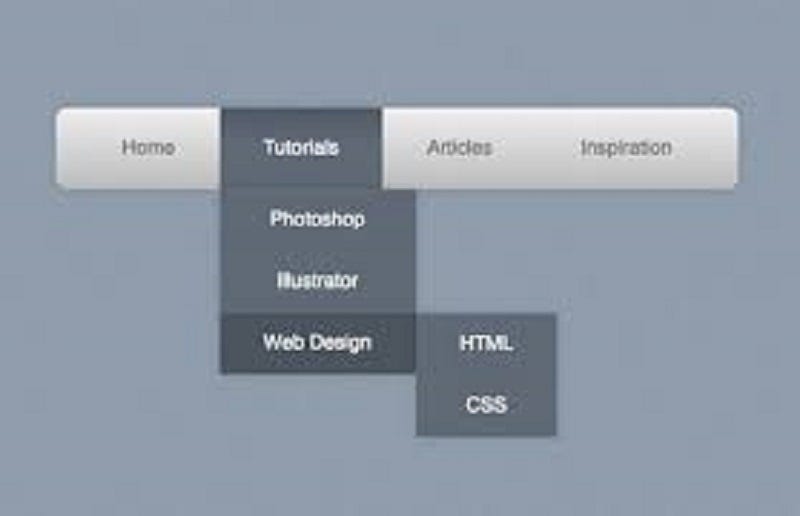In this slightly blurry image, you can see the top menu bar of a website with drop-down options. The main menu includes buttons labeled "Home," "Tutorials," "Articles," and "Inspiration." The menu bar is set against a light gray background with the main menu text appearing in a darker, possibly gray, font. The "Tutorials" menu is highlighted in dark blue, indicating it's selected, and it expands into a drop-down menu displaying options for "Photoshop," "Illustrator," and "Web Design" in white text against the dark blue background. The "Web Design" option is further highlighted, triggering an additional drop-down to the right that lists "HTML" and "CSS" in white text. The overall background of the image is a very light blue color, giving it a simple and clean aesthetic.